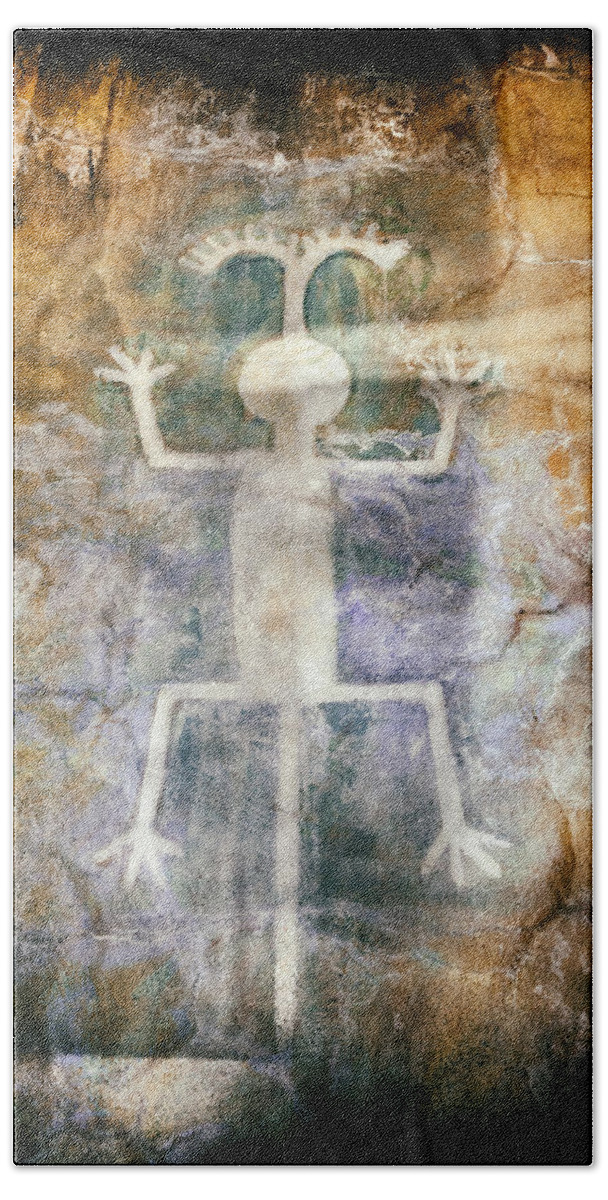The image depicts an ancient artwork on a weathered, mosaic-like cave wall. The wall's color transitions from dark black at the top, through shades of brown, green, and purple, returning to dark black at the bottom. The artwork itself is a profile outline of a lizard-like creature with a round head, featuring two long, antennae-like projections. The creature possesses two arms and two legs, each ending in four spread-out fingers or toes. It also has a long, straight tail and a bifurcated tongue extending from its head. The image appears lighter than the wall, with a darker outline accentuating the figure.